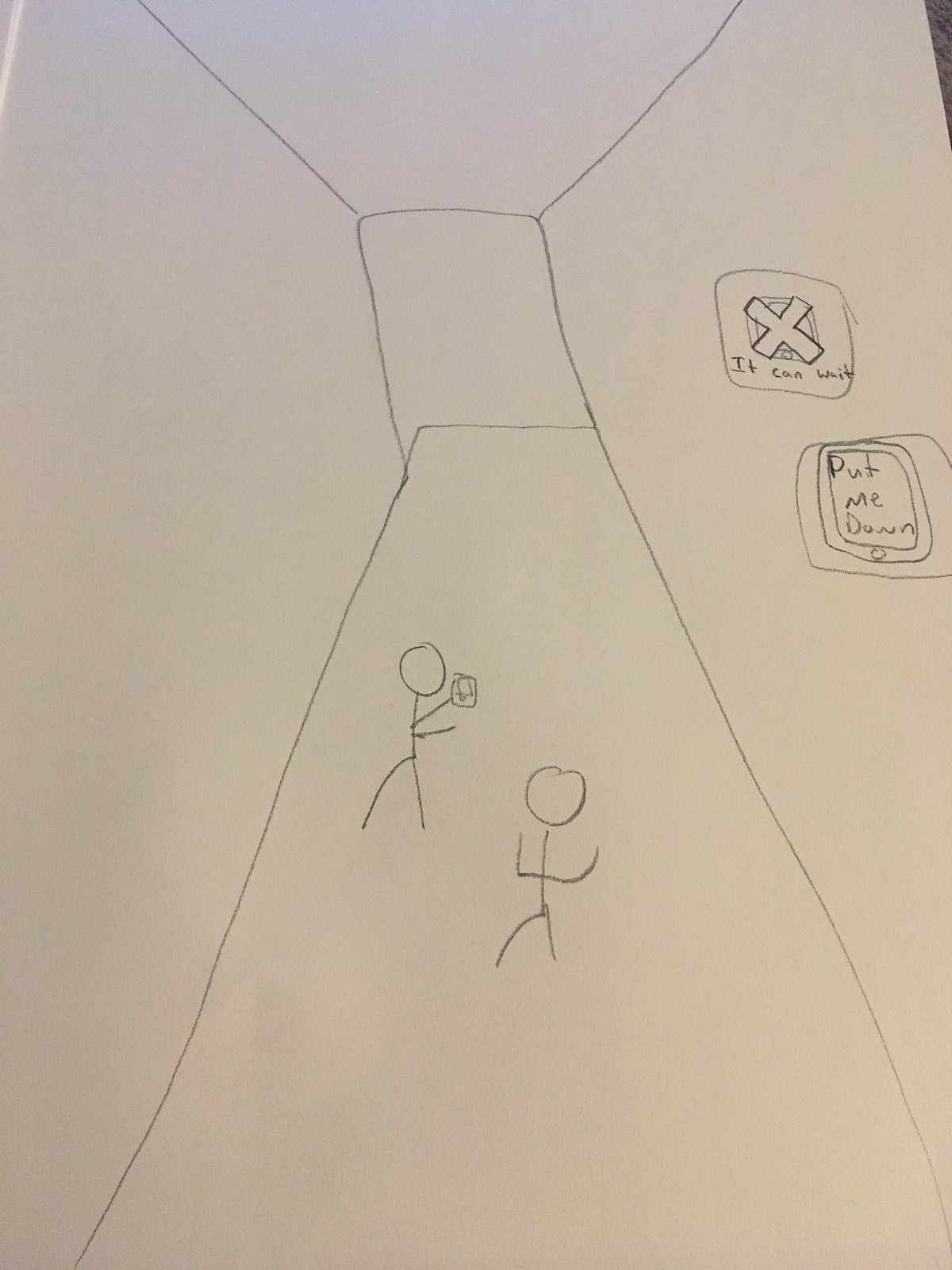This is a child's monochromatic pencil drawing on a white piece of paper, depicting two stick figures situated in a corridor with a distinct 3D perspective, where the hallway tilts towards the center and ends in a tiny back wall devoid of any doors or windows. The ceiling features lines radiating outward, enhancing the depth perception. One stick figure, on the left, holds a rectangular object, likely a phone, while pointing towards the right. The other stick figure on the right has its arms raised. Both figures lack facial features. On the right-hand side of the drawing, two signs are prominently displayed. The first sign, featuring a square with an X in the middle, is labeled "It can wait." The second sign, depicting a phone, carries the message "Put me down." This illustration emphasizes the encouragement to refrain from using phones. The upper right-hand corner of the image subtly reveals the brown surface on which the drawing was placed, while a lighter white line appears in the upper left-hand corner.